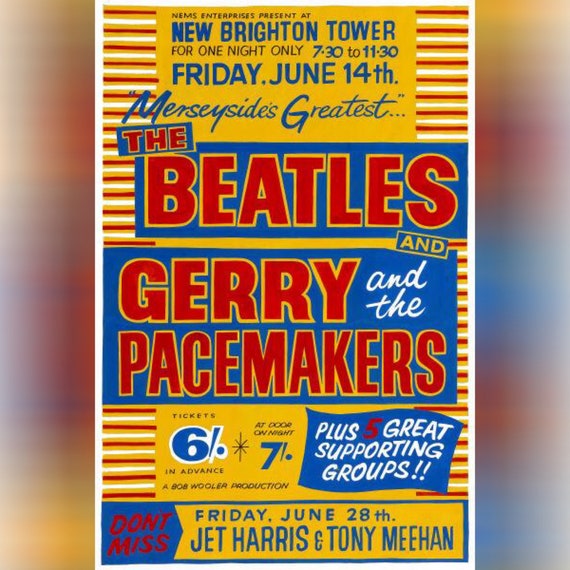The concert poster for an event at New Brighton Tower is vibrant with bold colors and intricate designs. The background features striking yellow, red, and white stripes, with text boxes in yellow and bright blue. At the very top, a yellow box with blue text reads, "Nemas Enterprises presents at New Brighton Tower for one night only, 7:30 to 11:30, Friday, June 14th, Merseyside's Greatest: the Beatles and Gerry and the Pacemakers." Details about ticket prices follow: "Tickets: 6.0 pounds in advance, 7.0 pounds at the door," indicated in yellow and bright blue text boxes with bold red and black fonts. A note at the bottom highlights additional performances: "Plus five great supporting groups," in a blue banner with white text, with the 'five' highlighted in red. Another blue banner declares, "Don't miss, Friday, June 28th: Jett Harris and Tony Meehan." The poster is a Bob Wooler production, emphasizing the significance and exclusivity of these events for music fans.